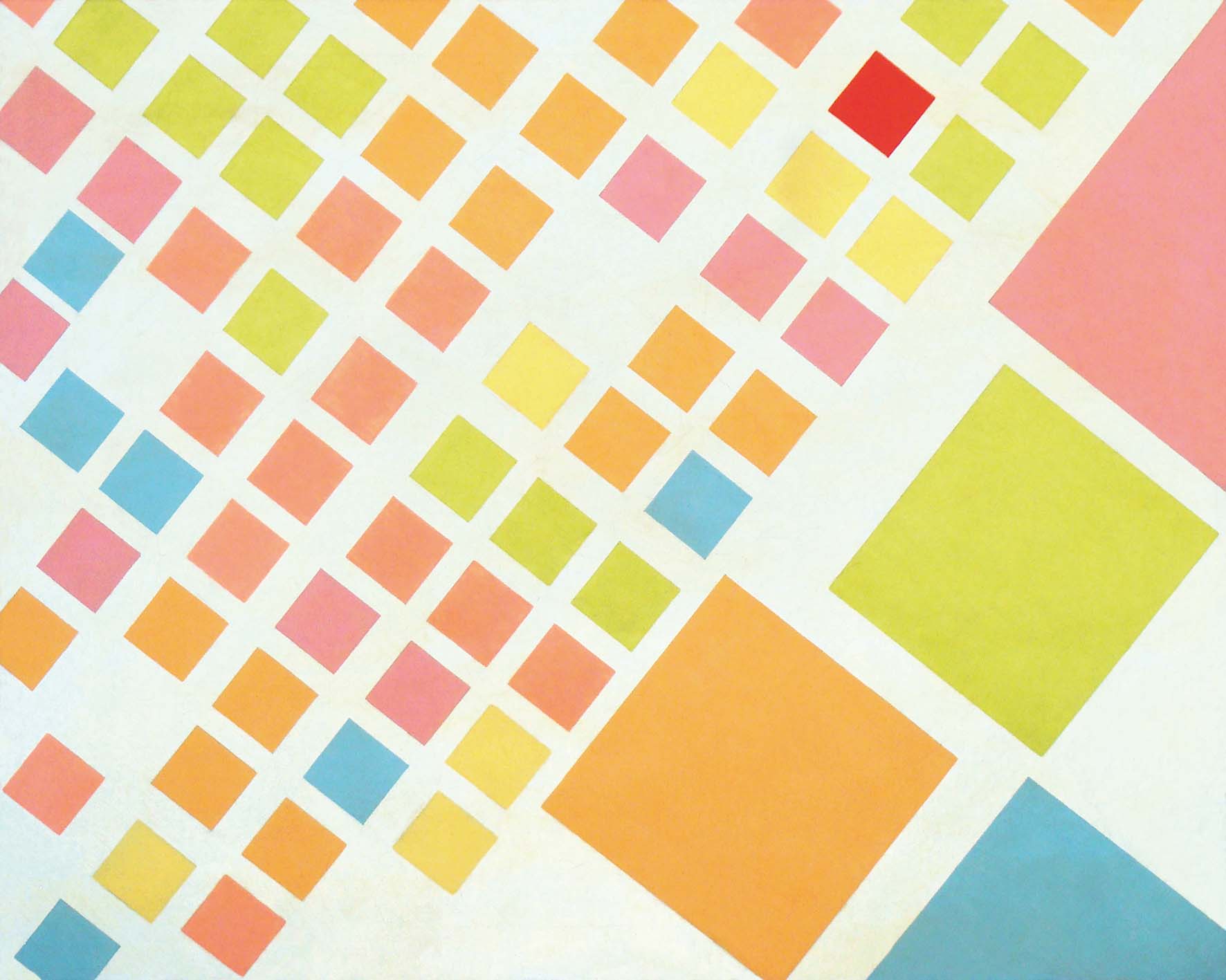The image showcases an abstract, Cubist-inspired design primarily composed of geometrical squares arranged meticulously against a white background. The overall structure forms a large square, which is subdivided into smaller squares that transition in size from the left to the right. On the left side, there is a dense array of smaller squares placed at a diagonal angle, creating a visually engaging pattern that gradually decreases in density from the bottom-left to the top-right corner. These small squares come in various soft, warm tones including shades of light greenish-yellow, pink, light blue, and orange. Notably, there's a lone, vivid red square strategically placed among them, standing out due to its rich hue.

As you move towards the right side of the image, the squares increase significantly in size, with about four large squares dominating this section. These larger squares are spaced evenly with white negative space between them, enhancing the optical effect of the design. The colors of these larger squares include a light olive, orange, pink-red, and blue. Despite the vivid and varied colors, there is no text, date, or signature present on the image, leaving its medium—whether watercolor, painting, or computer-generated—ambiguous. The deliberate arrangement of squares and the use of negative space give the piece a modern, almost logo-like quality while also resembling a piece of contemporary art.